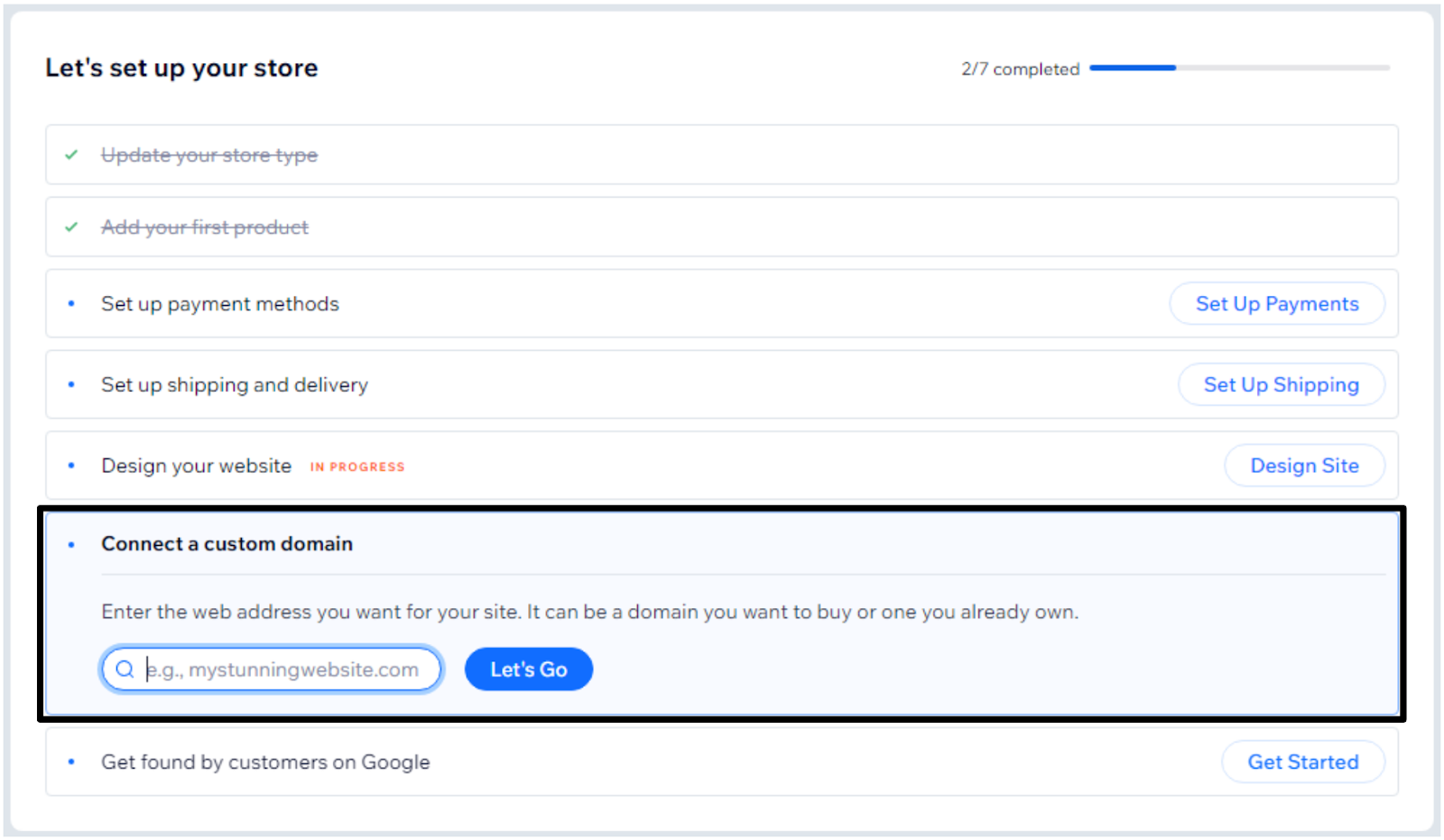A screenshot displays the backend interface of an online store setup on a computer monitor. The central focus is a gray-outlined window with a white background. In the upper left corner of this window, bold black text declares, "Let's set up your store." On the right-hand side of the window, progress is indicated by a "2 out of 7 completed" marker and a blue progress bar showing approximately 25% completion.

Below this progress marker is a checklist detailing tasks that have been completed and those that are pending. The first two tasks, "Update your store type" and "Add your first product," each have a strikethrough line and a green checkmark to their left, signifying their completion. Three tasks remain, each indicated by a blue dot on the left: "Set up payment methods," "Set up shipping and delivery," and "Design your website." To the right of these tasks, an orange text label displays "In progress."

At the bottom of the window is a black-outlined box with the heading "Connect a custom domain." Inside, instructions read: "Enter the web address you want for your site. It can be a domain you want to buy or one you already own," accompanied by a search box. To the right of this box is a blue button with the white text "Let's go."

At the very bottom of the list, another task marked with a blue dot reads, "Get found by customers on Google," followed by a blue button on the right with the label "Get started."

This structured and informative interface guides the user through the essential steps necessary to fully set up their online store.